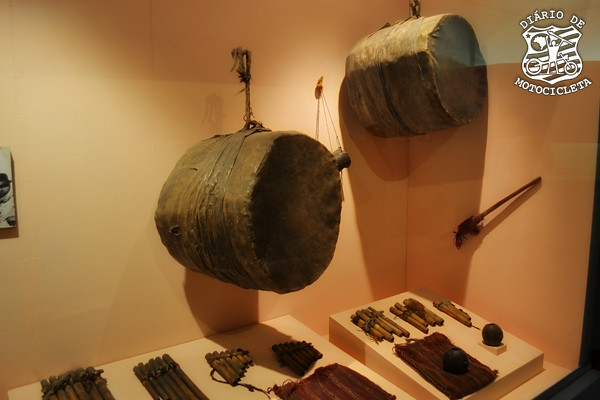This landscape-format, color photograph captures a museum display that showcases an array of ancient musical artifacts behind a reflective glass pane. The enclosure itself is light orange or peach colored, providing a warm backdrop to the collection. Prominently displayed on the upper part of the wall are two large, round drums, likely made from animal hide, which exhibit a well-worn, aged appearance. Lower down are several flutes, notably pan flutes, arranged in a line. These flutes, made from cylindrical wooden tubes with open ends, vary in size, becoming smaller from left to right and are held together by rope. The wooden cylinders are dark brown and show signs of significant wear, suggesting their antiquity. Additionally, there are small ball-like objects that could be shaken to produce sound, possibly filled with stones. These musical instruments, ranging from weathered drums to rustic flutes, highlight the diverse craftsmanship of ancient musical traditions.